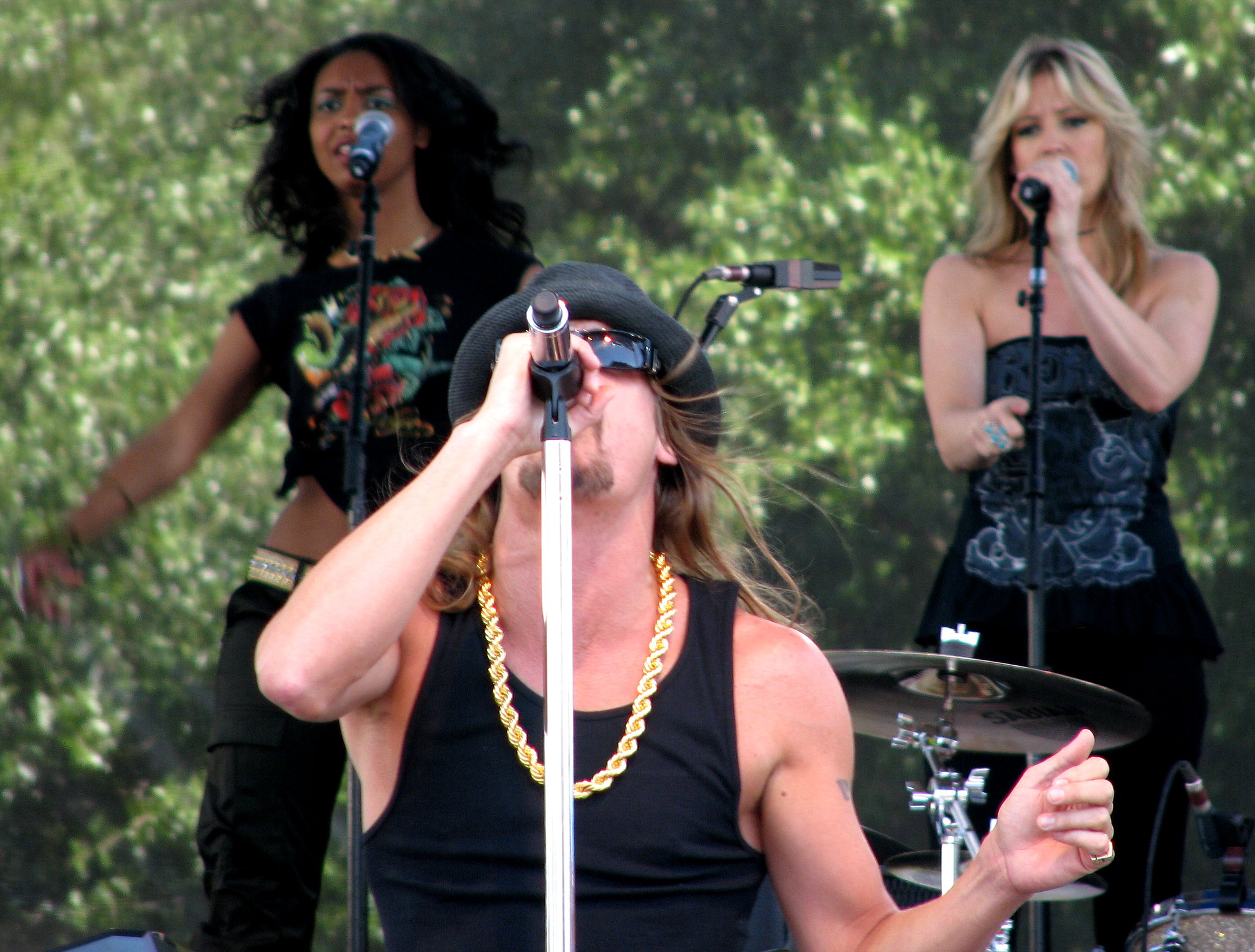The image captures singer and musician Kid Rock in an outdoor performance, surrounded by lush trees in the background. He stands center stage, passionately singing into a microphone. Kid Rock sports a black tank top that showcases a hefty gold chain around his neck. His distinct look is completed with a fedora hat and sunglasses, a goatee, and long, windswept, blondish-brown hair. Flanking him are two female singers. On his right stands a Caucasian woman with long, feathered blonde hair, wearing a strapless black top and black pants. On his left is an African American woman with dark hair, dressed in a black shirt featuring abstract blue and green artwork, along with black pants and a white belt. Both women hold microphones and are immersed in their performance. Behind them, part of a drum kit with cymbals is also visible, adding to the concert ambiance.